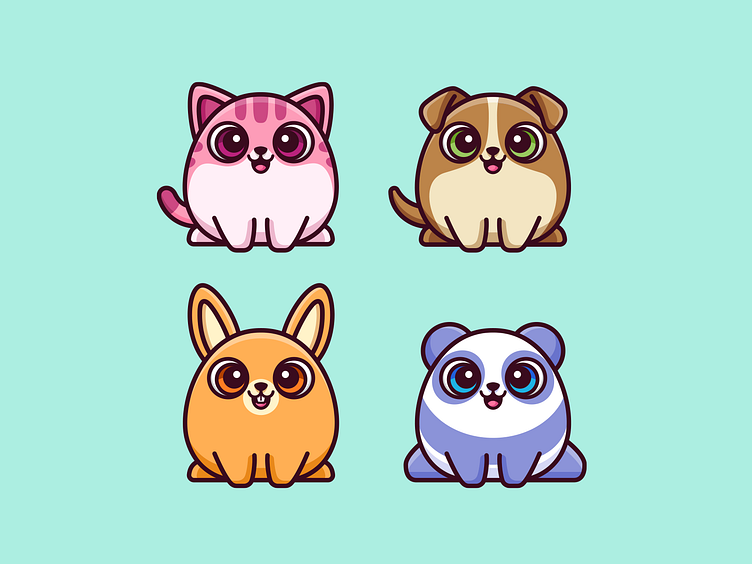This color illustration, set against a mint green background, features four cartoon-like, animated animal characters arranged in a two-by-two grid. In the top left corner, there's a round, smiling cat with pink shades on top, a lighter pink underbelly, pink stripes on its head, and purplish eyes, accented by its tiny short legs. Next to it, on the top right, sits a round, cheerful dog with big round green eyes, brown fur with a lighter beige underbody and face, flopped-forward ears, and small feet. On the bottom left, an orange bunny with orange eyes and a light brown tint, pink inside its long ears, and a slightly opened mouth to reveal two small teeth, is smiling. Finally, on the bottom right, there is a unique panda bear with a non-traditional blue and white coloring, bright blue eyes, a pink tongue, and a tiny nose, also displaying a cheerful expression. All the characters exude a very cute and adorable quality, highlighting their cartoon look against the clean mint green backdrop.